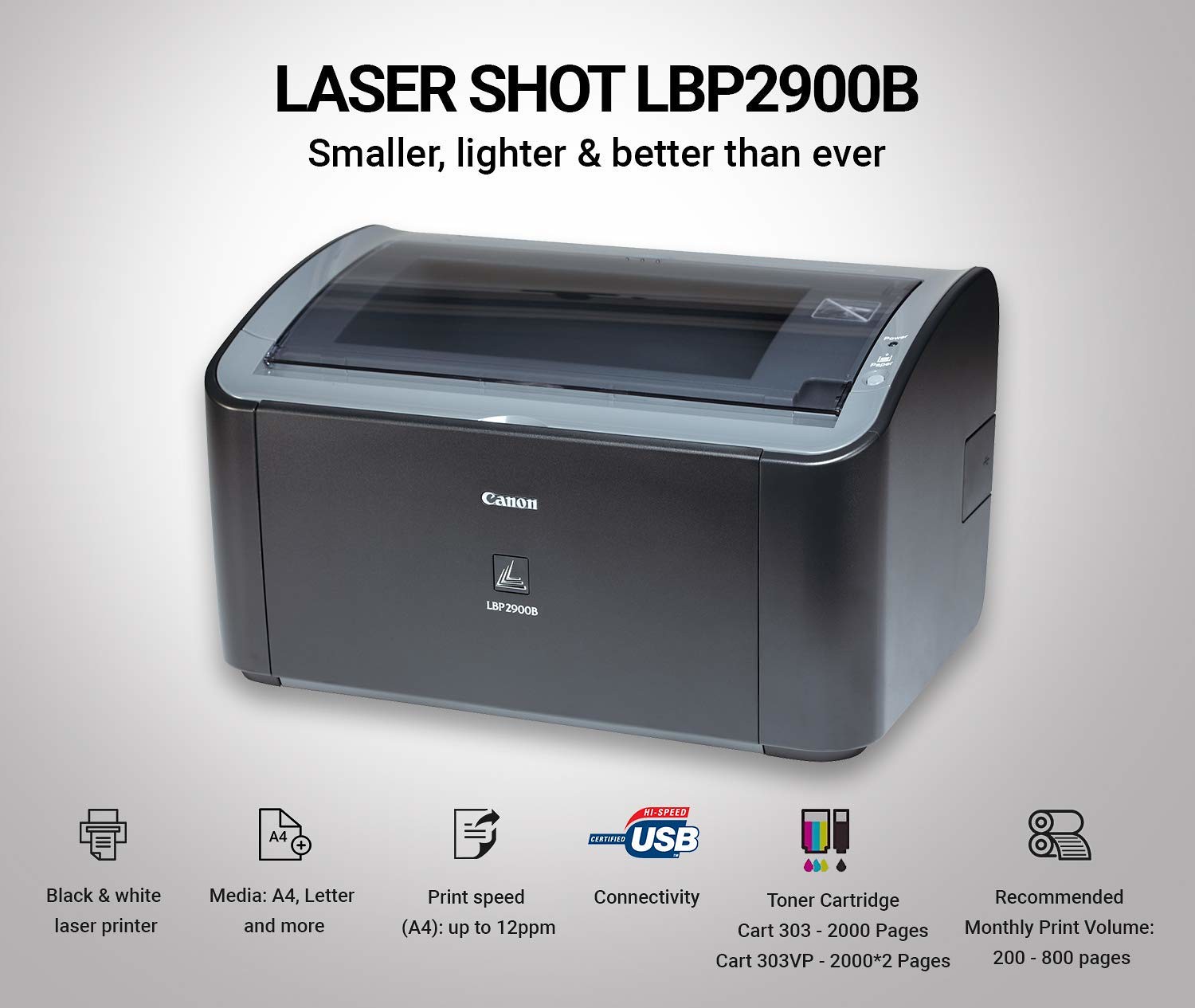The advertisement for the Canon LaserShot LBP 2900B features a sleek black and gray laser printer set against a grayish-white background. Prominent black text at the top reads "LaserShot LBP 2900B: Smaller, lighter, and better than ever," emphasizing the printer's improved features. The printer itself is shown in a slightly angled front view, with the Canon logo in white positioned centrally on its body.

Below the image of the printer, a series of icons and descriptive texts highlight its key specifications: it is a black and white laser printer, compatible with various media sizes including A4 and letters, and boasts a print speed of up to 12 pages per minute. Connectivity is supported via USB, illustrated by a blue-outlined USB symbol, and a high-speed red tag is also featured. The toner cartridge specifications are listed, indicating "cartridge 303 for up to 2000 pages" and "cartridge 303VP for up to 2000+ pages." Lastly, the recommended monthly print volume ranges between 200 to 800 pages. The overall layout and detailed descriptions clearly aim to showcase the printer's capabilities and suitability for different printing needs.